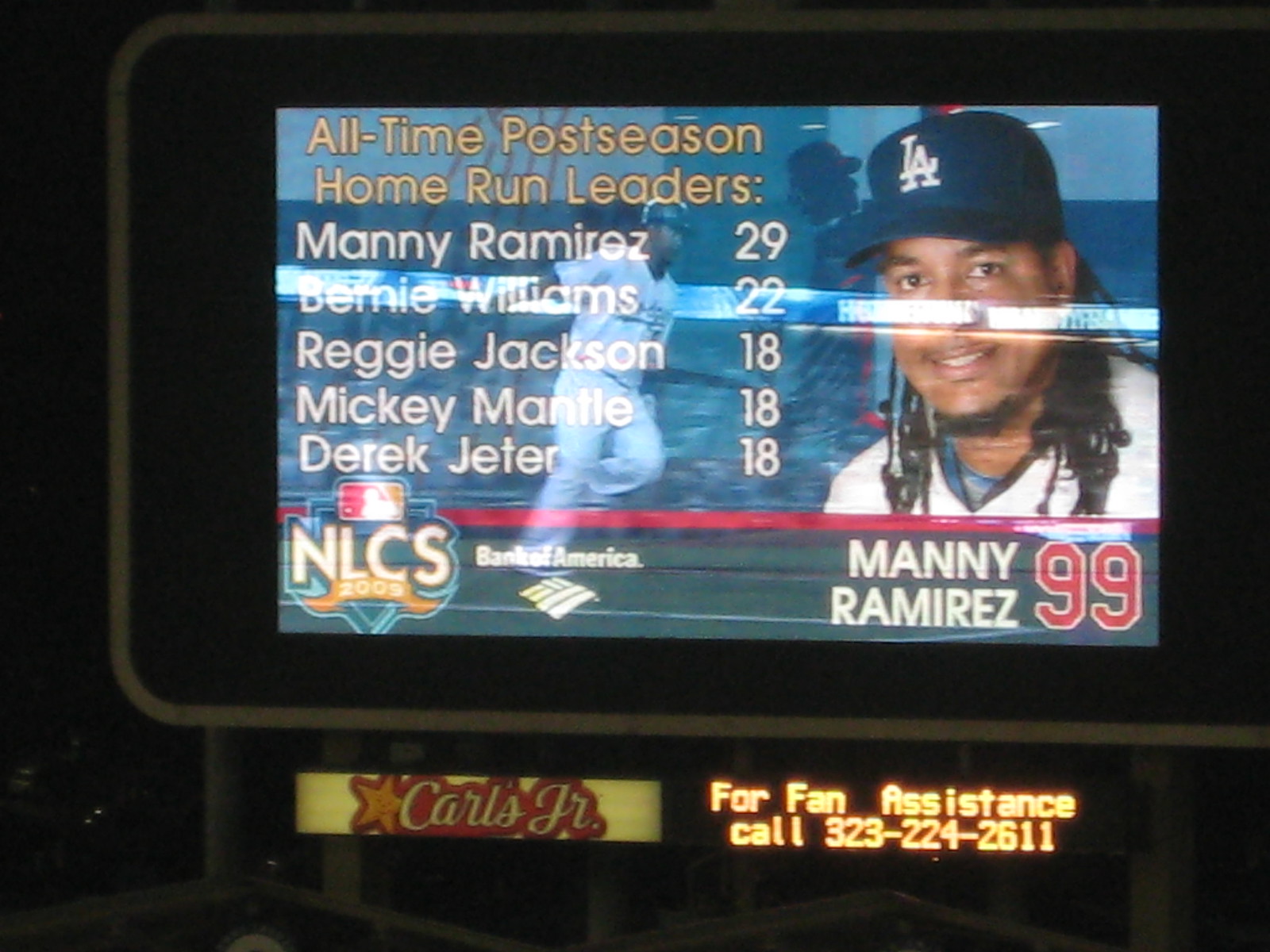The photograph captures a large digital monitor atop a building, resembling a billboard or an advertisement, at a nighttime baseball game, most likely viewed from the outfield. The screen prominently features the heading "All-Time Postseason Home Run Leaders" in the upper left corner, with a list of names and their respective home run totals: Manny Ramirez (29), Bernie Williams (22), Reggie Jackson (18), Mickey Mantle (18), and Derek Jeter (18). To the right of the text, there is a photograph of a black man with dreadlocks, identified as Manny Ramirez, wearing a white or blue "LA" baseball cap and a white uniform. Below his image, the text reads "Manny Ramirez 99." In the lower left-hand corner, the screen mentions "NLCS 2009" alongside the Bank of America logo. Additionally, directly below this digital monitor, there's a Carl's Jr. sign, and adjacent to that, bright neon letters display a message for fan assistance with the number "323-224-2611" for contact. The dark background indicates that this event is occurring at night.